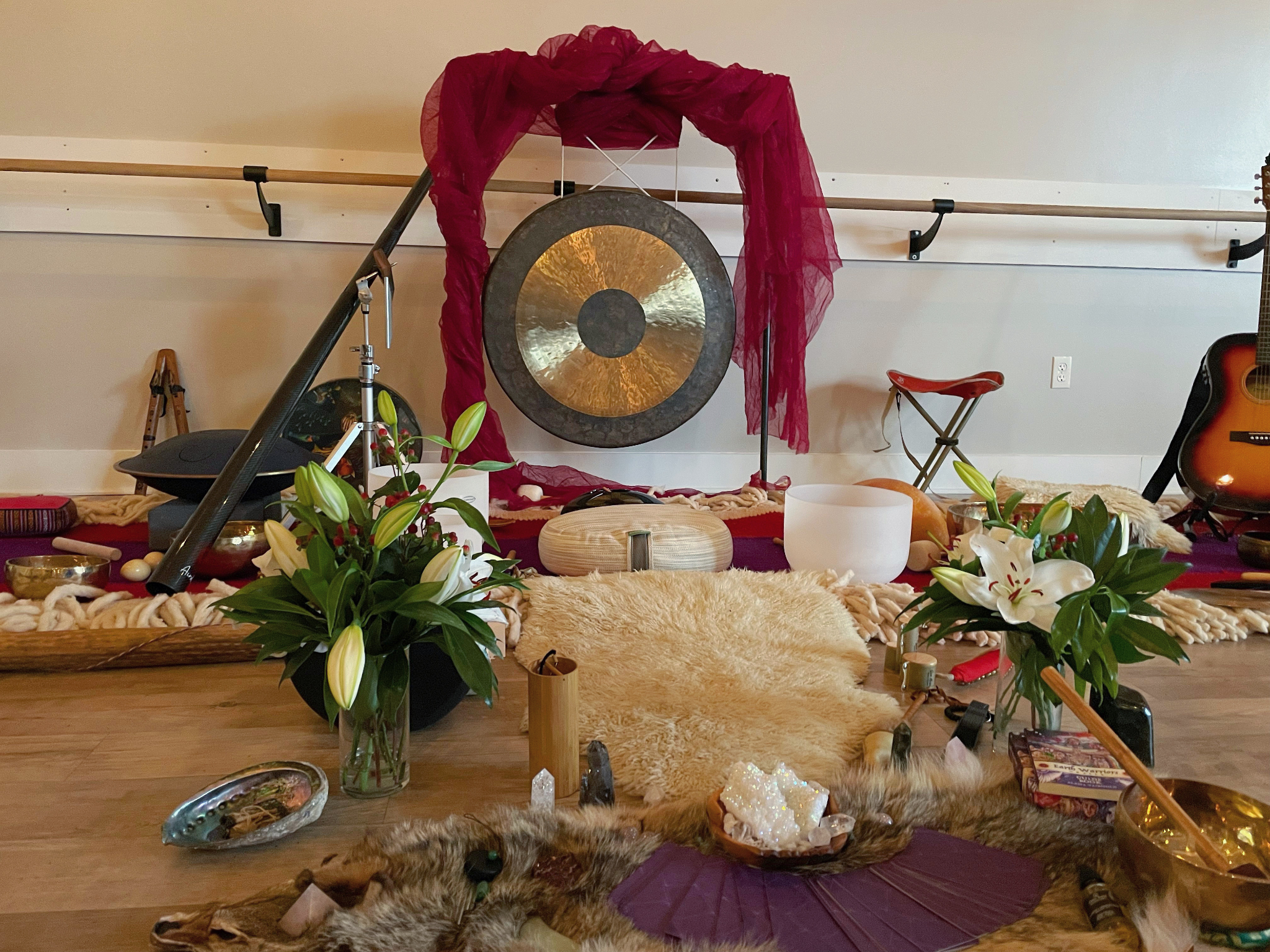The photograph depicts an intricately arranged indoor stage setup centered around a large gold and black gong mounted on a black frame, which is partially concealed by a vibrant red shawl. The gong sits against a light gray wall adorned with a brown wooden railing, reminiscent of a ballet studio's handrail. In the foreground, a plush cream-colored fur rug and a colorful carpet create a cozy, inviting scene. Scattered across the carpet are various musical instruments, including a long flute, a unique double-barreled flute, and an acoustic guitar positioned in a stand to the right. Additional items, like white lily plants in glass vases, a polished abalone shell, and an assortment of wooden bowls and spoons, contribute to the rich, ritualistic atmosphere. This well-composed tableau, featuring both musical and decorative elements, seems to evoke a serene and ceremonial vibe.